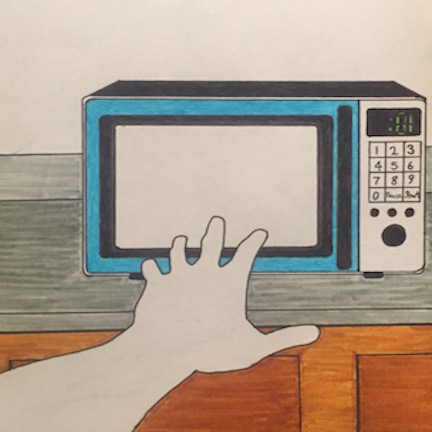This detailed drawing of a microwave oven features it prominently positioned slightly to the right of center on a gray countertop with a matching gray backsplash. The scene is set against a cream-colored background that extends to the white walls beyond. The microwave itself has a sleek design with a black top and black handle. Its front is accentuated by a turquoise frame surrounding a black window, through which a white inner compartment is depicted, likely signifying the viewing window. 

A thin silver border separates the top black portion from the turquoise front. On the right side of the microwave, there's a digital display showing "01" in a vibrant yellow or green, indicating one second remaining. Below the display are four rows of three cream-colored squares with black digits ranging from 1 to 9 and additional text on the bottom row. Beneath these are three small black circles and one larger black circle, aligning perfectly under the square columns above.

In the foreground, from the bottom left corner of the image, a left arm rendered in white with black outlines is reaching towards the microwave. The four fingers are extended and nearly touching the appliance, with the thumb positioned below the countertop. The scene captures the countertop’s gray surface supported by wooden cabinets in a medium warm brown tone with simple, unembellished black-trimmed rectangles. The image's detailed coloring and pen outlines provide a vivid, almost tactile sense of the scene and action.